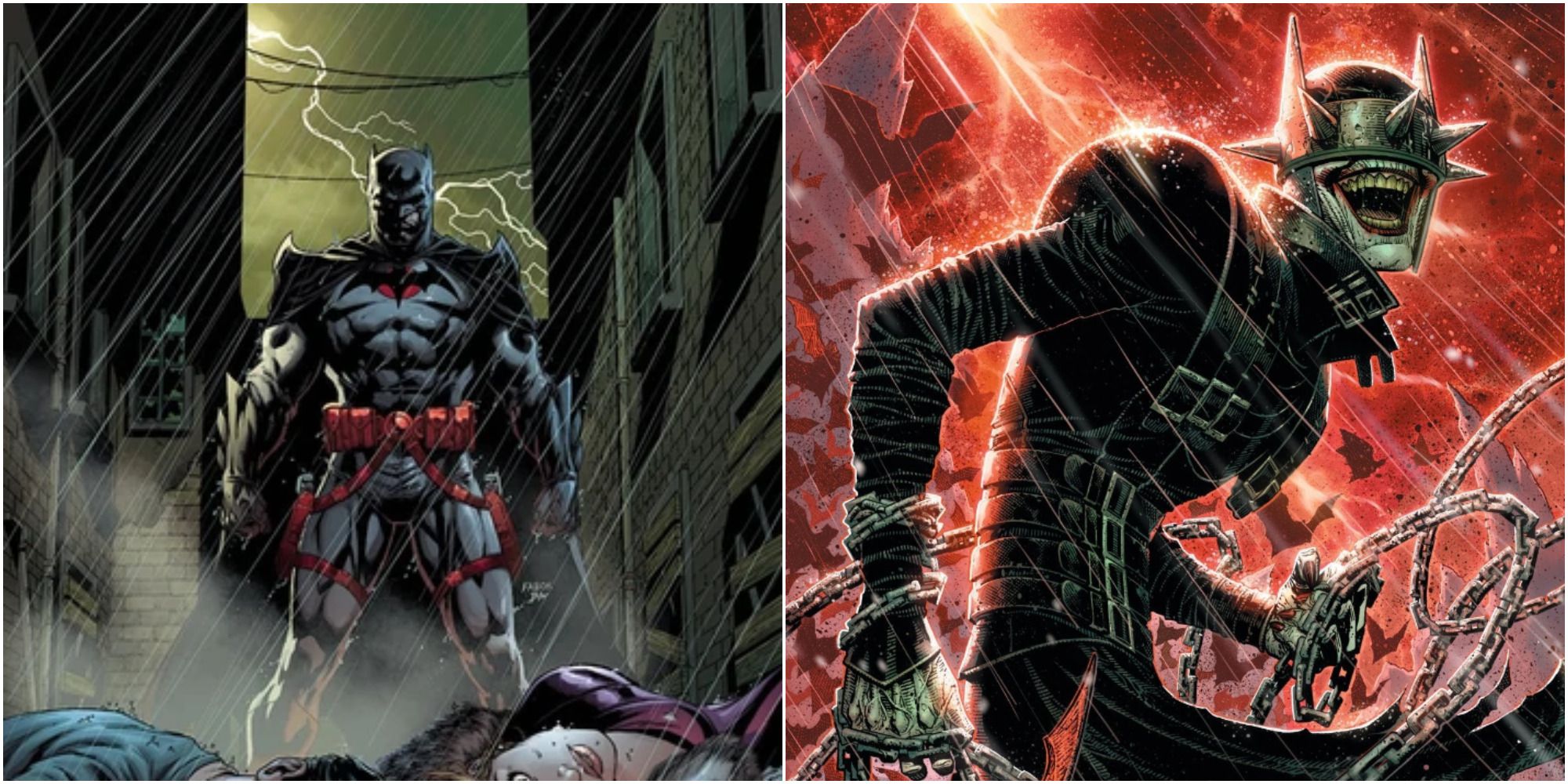The image is divided into two distinct halves, showcasing illustrated depictions related to Batman. The left half features Batman himself, clad in a grey and black costume adorned with the signature pointed mask. Notably, he sports a red belt that extends into garters around his legs. Batman stands resolutely in the rain, framed by very dark buildings that suggest an ominous alleyway setting. A dramatic streak of lightning illuminates the sky behind him. On the ground before Batman lie two figures: a woman with brown hair in a purple dress and a man with short black hair wearing a blue shirt, both appearing lifeless.

The right half of the image presents a character that appears to be a villain. He is dressed in a menacing black trench coat, with chains ominously wrapped around his hands. His helmet is particularly striking, featuring a visor adorned with spikes covering his eyes. The backdrop is a vivid red, accentuated by a bolt of lightning, adding to the intense and foreboding atmosphere of this half of the illustration.